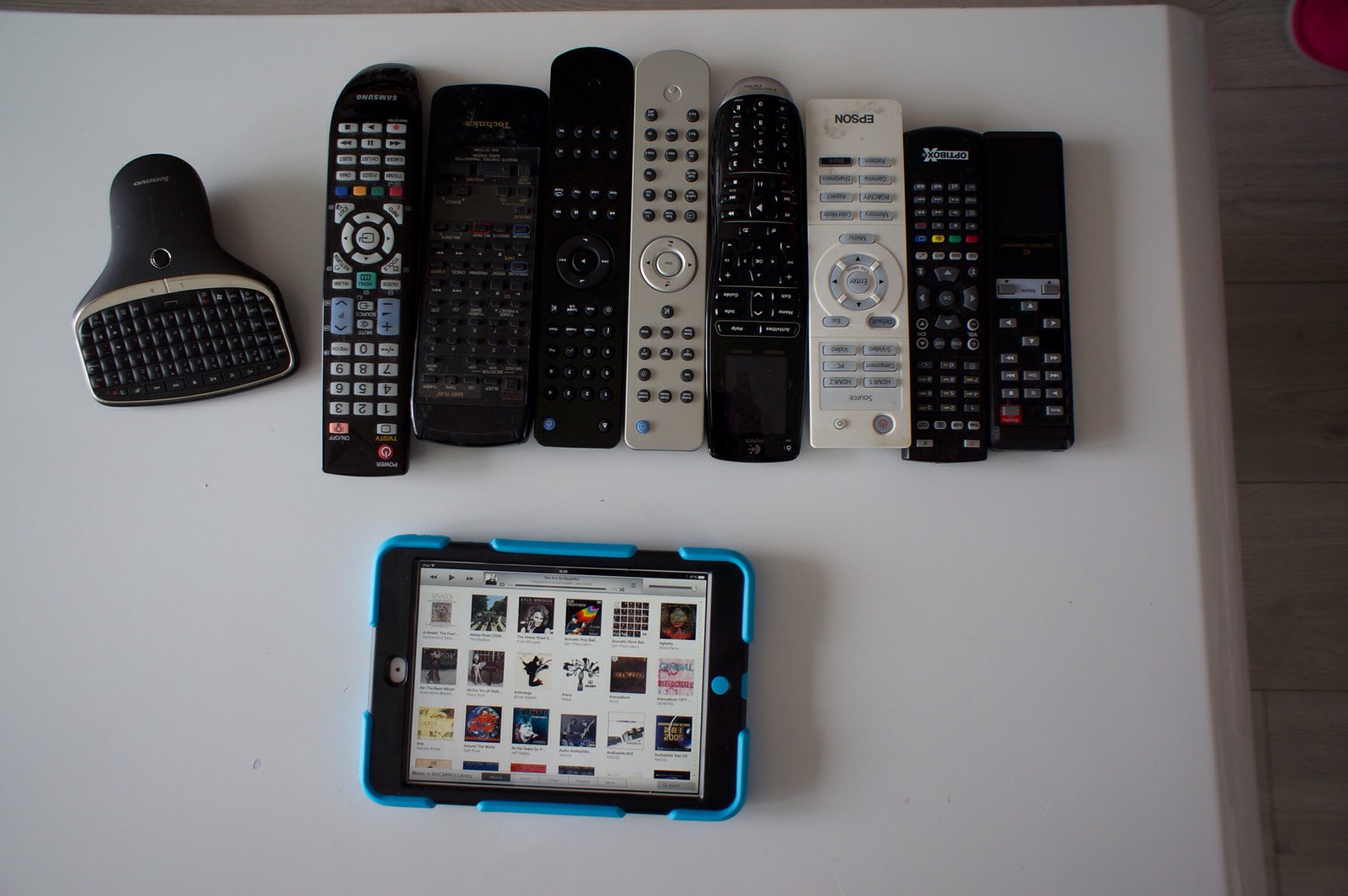The image shows eight remote controls of various sizes and colors, predominantly black, with one white and one gray remote. They are neatly lined up next to each other on a white surface. To the left of the remotes is an unidentifiable device featuring a keypad and likely lights up when a button is pressed. Underneath the remotes lies a tablet, possibly an older iPad model, enclosed in an aqua-colored case. The tablet's screen displays multiple icons or pictures arranged in a grid.